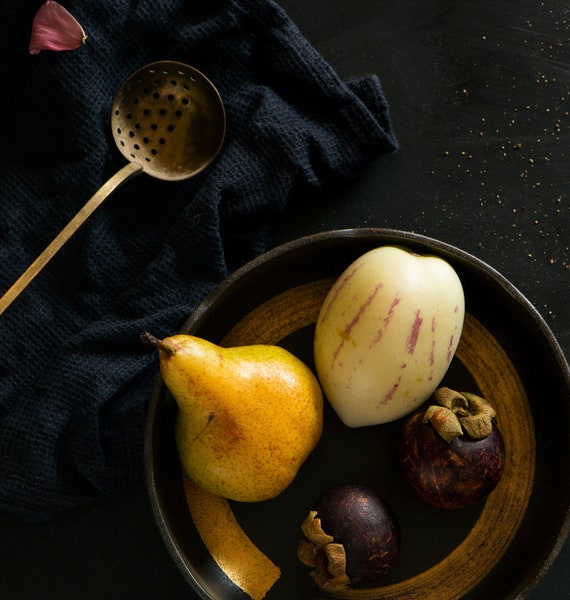The photograph features a dimly lit kitchen counter or table surface, predominantly black with white speckles, possibly a tablecloth. In the top right corner, light brown or yellow crumbs are scattered. Atop a dark navy blue woven towel on the left side of the image rests an old, bronze or gold ladle with half its surface solid and the other half perforated, functioning like a strainer. Nearby, a singular dark pink rose petal lies on the towel.

In the bottom right corner of the image, there is a black wooden bowl with a gold circular interior band. Inside the bowl are several pieces of fruit: a blemished yellow pear with some brown spots on the left, a whitish fruit with faint purple or red streaks resembling a melon or gourd, and two dark purple fruits with brownish tops, possibly figs or beets. The overall ambiance of the image is quite dark, emphasizing the contrasting colors of the fruit and the subtle details on the surface.